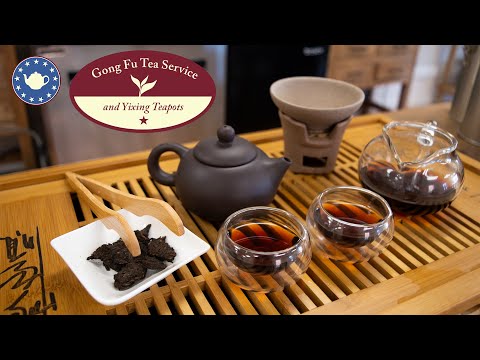The image is a photograph featuring a Gong Fu tea service setup. At the top left corner, there is a blue circle adorned with white stars and a white kettle at its center. Nearby is a prominent oval outlined in red; the top half of the oval has a deep maroon background with white text reading "Gung Fu Tea Service," while the bottom half is cream-colored with maroon text that says "And Yixing Teapots." Below these elements, the tea setup is displayed on a wooden tray with slats running horizontally and vertically, creating a gridded pattern. The main components of the tea set include a solid, dark gray Yixing teapot and a matching gray bowl, both stone-like in appearance. To their right sits a glass pitcher containing a small amount of amber liquid, presumably tea. In front of the teapot, there are two round glass teacups, each filled with the same amber liquid. To the left, there's a small square white tray holding some indistinguishable black objects, possibly tea leaves or tools, accompanied by wooden tongs. The overall setting is framed by thick black borders at the top and bottom, giving the image a formal and polished appearance.